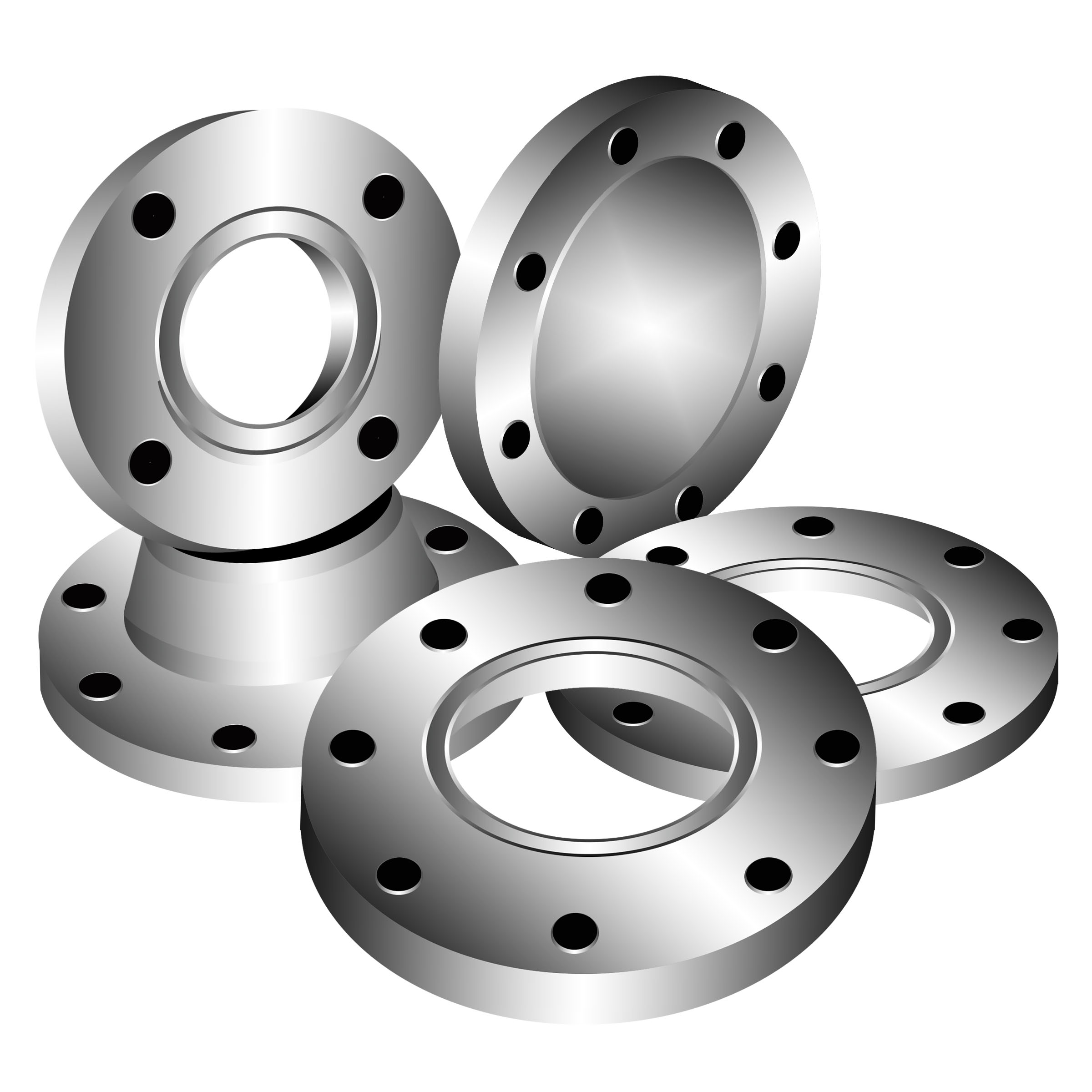The image features several large, round silver-colored objects set against a plain white background. These objects resemble automotive parts or washers and vary slightly in design. All are circular with either solid or hollow centers, and they are punctuated by small black dots around their edges. 

In the top left corner, one object with a hollow center and four small black holes around its edge is balanced atop another lying flat. The latter has numerous small black circles cut out around its perimeter. 

In the foreground, a large circular object with a hollow center and eight small black holes around its edge is partially lying on top of another identical object that is flat on the ground.

In the upper right corner stands a circular object with a solid center and eight black dots around its edge. This collection of metallic circles, with their repetitive patterns of holes and varied central designs, is sharply defined against the stark white backdrop.